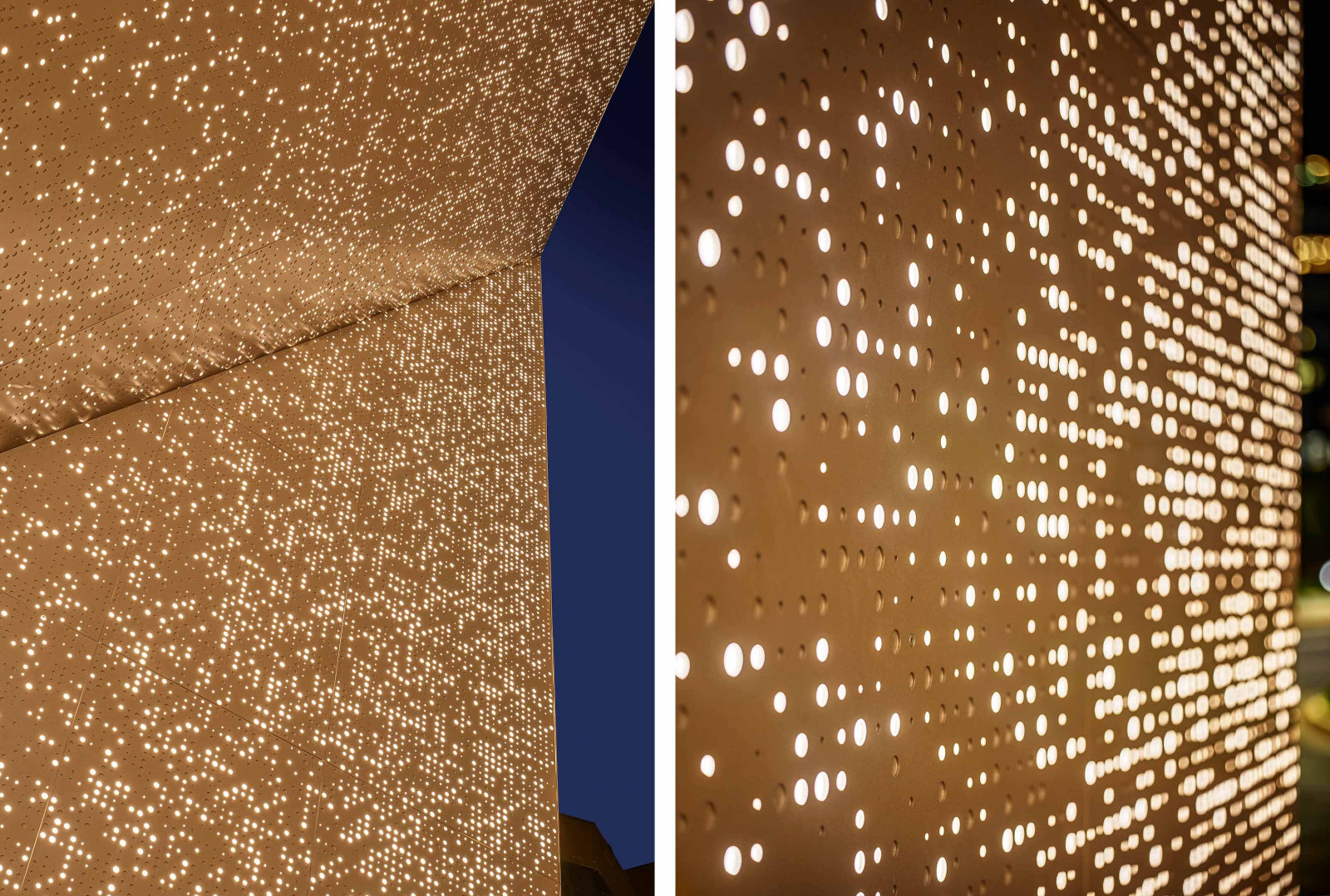The image captures a close-up of a large, gold-colored structure, potentially an art installation or building, situated outdoors at night. The structure features numerous holes, some illuminated by small white lights, creating a striking visual against the gold surface. On the left side of the image, the gold appears darker and dotted with a multitude of tiny, glowing white lights, interspersed with more holes that do not have lights. This section also reveals a background of deep blue, reminiscent of the night sky. To the right, the same structure seems magnified, showing larger, less frequent holes, many of which also contain white lights. The illuminated holes on both sides create a random, abstract pattern against the gold surface. In the background, additional building lights contribute to the night-time setting, and indentations on the structure suggest an irregular texture or design.